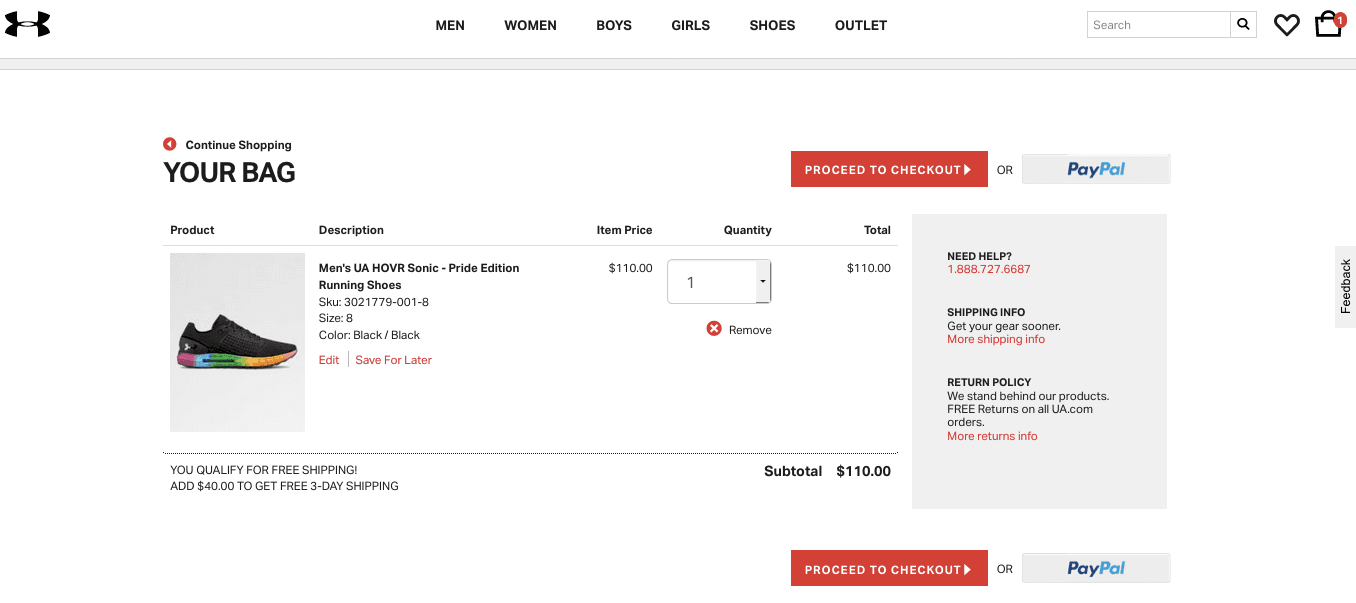Screenshot of an Under Armour online shopping cart displaying a pair of shoes. 

In the upper left corner, the black Under Armour logo is prominently visible. At the top, navigation options are listed: Men, Women, Boys, Girls, Shoes, and Outlet. The upper right corner features a search bar, a heart icon, and a shopping bag icon with a red circle indicating 1 item inside.

Below the navigation bar, several action prompts are available: Continue Shopping, Your Bag, Proceed to Checkout, and PayPal. The main section is divided into columns labeled Product Description, Item Price, Quantity, and Total.

The product displayed is a pair of black shoes with a vibrant, rainbow-colored sole. The detailed description reads: "Men's UA HOVR Sonic Pride Edition Running Shoes, SKU 3021779-001-8, Size 8, Color: Black." Options for the product include Edit or Save for Later. The item price is listed at $110, with a quantity of 1 and a Remove button. The total cost for the shoes is $110.

A message states that the order qualifies for free shipping, and an additional $40 purchase would qualify for free 3-day shipping. The subtotal is $110.

Additional customer service information includes: "Need Help? 1.888.727.6687," links for Ship Info, Get Your Gear Sooner, More Shipping Info, Return Policy, We Stand Behind Our Products, Free Returns on All UA.com Orders, and More Returns Info. The screen also provides final options to Proceed to Checkout or use PayPal.